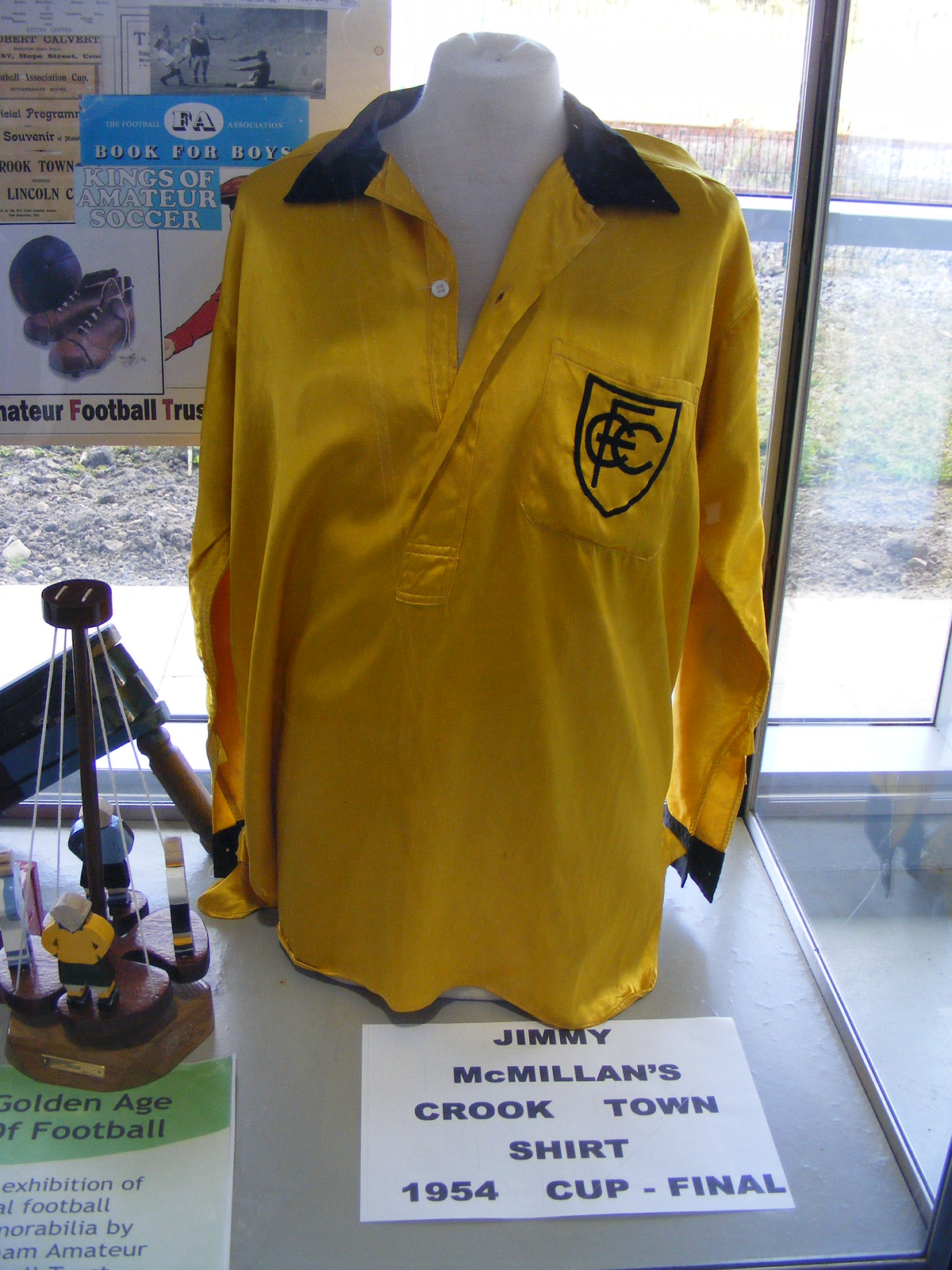This is a detailed photograph taken indoors, probably in a sports museum or a memorabilia shop, focusing on a display case showcasing soccer artifacts. The central feature is a mannequin bust dressed in a yellow, long-sleeve soccer jersey with a black collar and an open one-button pocket. The left chest pocket of the shirt bears the FCC logo. Beneath the shirt, a white piece of paper announces, "Jimmy McMillan's Crooktown 1954 Cup Final shirt," indicating the shirt's historical significance. To the left of the image, there is a background with a green section carrying black text and a white section with black text, promoting an exhibition titled "Golden Age of Football, Exhibition of Football Memorabilia by Ann Amacher." In the window behind the shirt display, signs can be seen, including one that reads "Book for Boys, Kings of Amateur Soccer, Amateur Football Trust," alongside an illustration of a pair of shoes. Additionally, there seems to be a wooden toy or mobile to the left of the shirt, accompanied by its own informational paper.